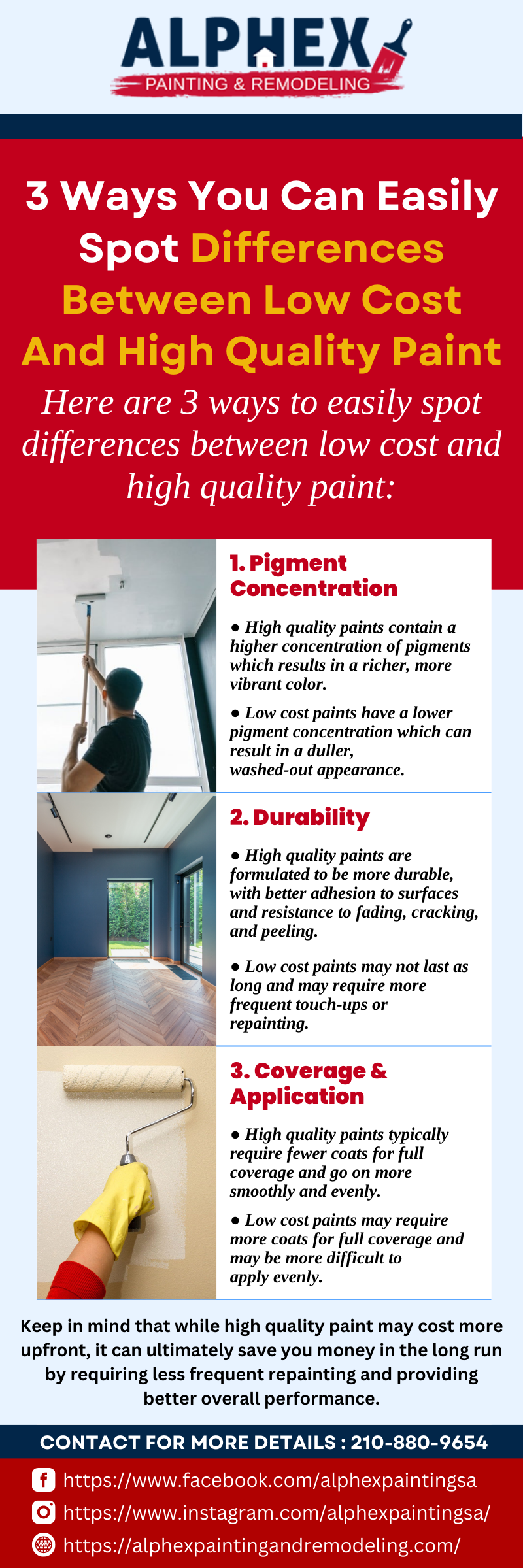This digital advertisement for Alphax Painting and Remodeling provides detailed guidance on how to distinguish between low-cost and high-quality paint. The ad header features "Alphax Painting and Remodeling" in dark blue text on a white background, with "painting and remodeling" in white text set against a brush stroke of paint. Below this, a red square highlights the main topic: "Three Ways You Can Easily Spot Differences Between Low-Cost and High-Quality Paint."

The advertisement breaks down the comparisons into three categories, each supported with a photograph for clarity:

1. **Pigment Concentration**: High-quality paints have a higher concentration of pigments, resulting in richer and more vibrant colors, whereas low-cost paints have less pigment, leading to a duller appearance. The accompanying image shows someone painting a roof, demonstrating the importance of pigment in achieving a consistent hue.

2. **Durability**: High-quality paints offer better adhesion, resisting fading, cracking, and peeling, thus lasting longer. Low-cost paints, on the other hand, may require frequent touch-ups. This concept is illustrated with a photo of an empty interior room, showcasing the lasting finish of high-quality paint.

3. **Coverage and Application**: High-quality paints typically require fewer coats for full coverage and are easier to apply smoothly and evenly. In contrast, low-cost paints may necessitate multiple coats and can be more challenging to apply. A close-up image of a gloved hand painting a wall emphasizes the ease of application with high-quality paint.

Additional information at the bottom of the ad reminds consumers that while high-quality paint may have a higher upfront cost, it can save money over time due to its longevity and fewer maintenance requirements. Contact details, including a phone number, and links to Alphax's Facebook, Instagram, and website, are provided for further inquiries.